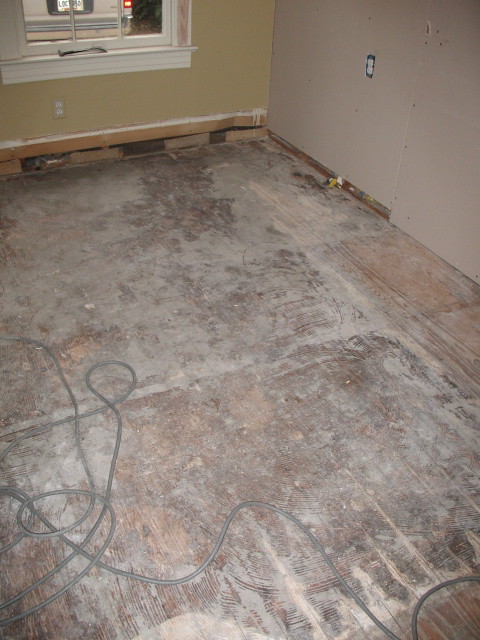The photograph captures an indoor scene of a room in the midst of renovation. The most noticeable feature is the bare, dirty subfloor, which appears to be raw plywood. Any former carpeting has been removed, revealing a floor cluttered with debris. A gray cord snakes from the left and winds towards the bottom right, adding to the disarray.

The room's walls show signs of ongoing work. The left wall is light tan and is missing its baseboard trim, with exposed wood visible where the trim once was. A new electrical outlet is installed but lacks its cover plate. Adjacent to this, a window with three panes remains intact, and through it, the rear end of a car with its backup lights on is visible.

The right wall features a mix of gray and cream hues, also missing its baseboard trim. Visible wood fragments are scattered along the base of the wall. Another electrical outlet, this one with its cover plate, contrasts with the incomplete look of the rest of the room. This photograph captures a space that is clearly under transformation, hinting at an ongoing renovation or restoration project.